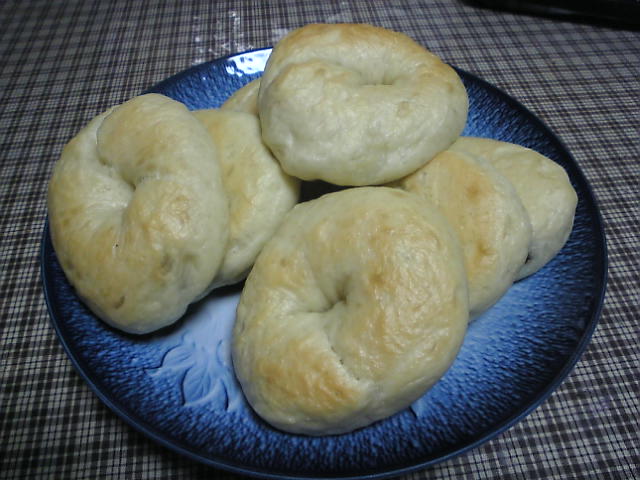The vibrant photograph showcases a beautifully arranged plate of what appear to be homemade bagels, each one unique in shape and size, indicating their artisanal nature. The bagels, seven in total, are stacked in a somewhat haphazard yet charming manner, displaying a light beige crust that suggests a gentle bake rather than a deeply toasted finish. These plain bagels lack any visible seasoning and show the classic ring shape, though some are more imperfect than others, adding to their homemade appeal.

They rest on a striking blue ceramic plate, adorned with a textured, pearlized leaf pattern, where the edges are a darker blue that transitions to a lighter blue towards the center, which is nearly white. This plate catches the light in a way that reflects a subtle sheen, amplifying its intricate design. The entire composition is set atop a dark blue and white plaid tablecloth that is covered with a clear protective layer, ensuring that the setup remains pristine. The photograph is elegantly simple, with the focus firmly on the inviting, fluffy bagels and the intricate, visually appealing plate on which they are carefully arranged.